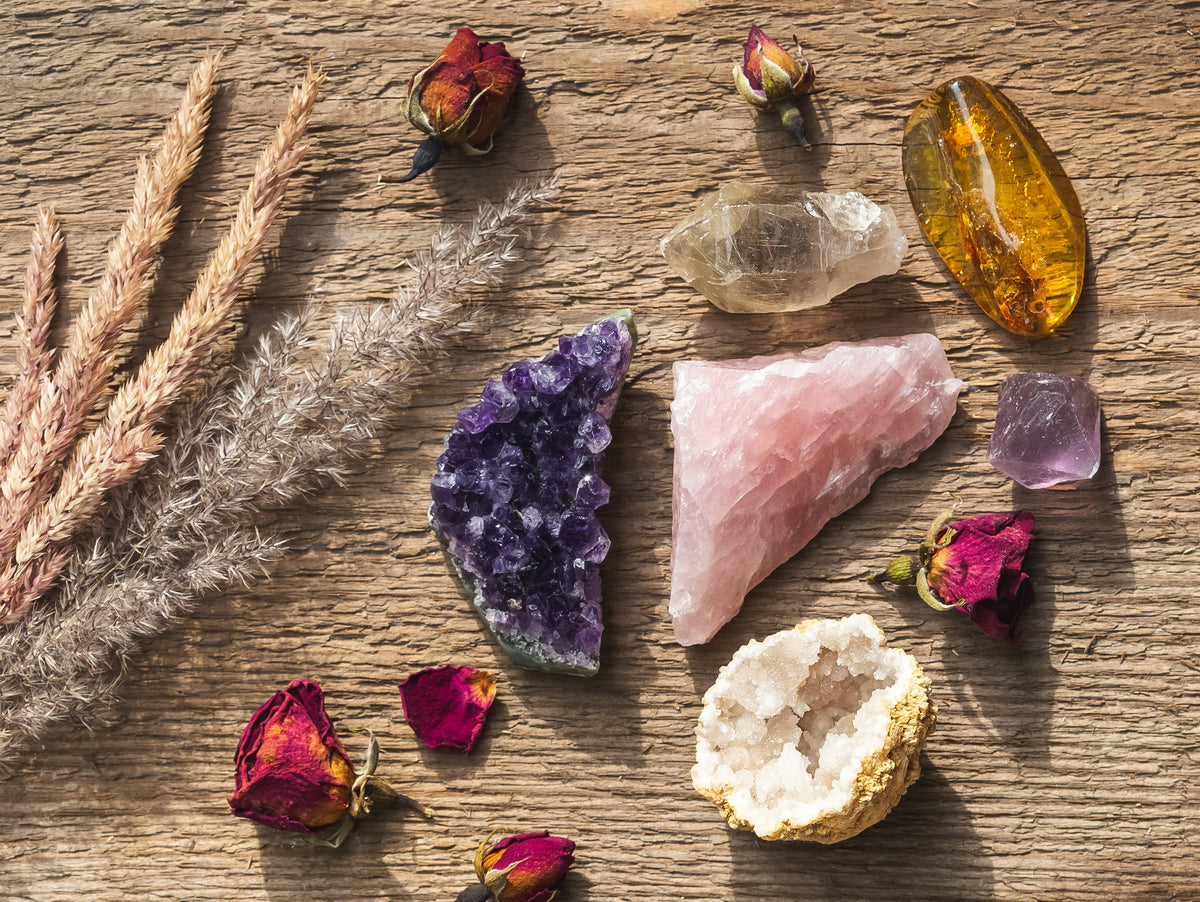The image displays a meticulously arranged collection of natural objects on a rough, light tan wooden surface, possibly a bench or log. On the left side, there are stalks, one resembling wheat and another with a more feathery appearance, both in natural beige and silvery hues. Dried orange roses are strategically placed at the top and bottom, adding a touch of aged elegance. Among these elements are various crystals: a striking purple crystal, a glistening geode, a piece of pink quartz, a neutral clear stone, a warm piece of amber, and another purple stone. The arrangement is artfully enhanced by the scattered dried roses and fronds, creating a visually appealing blend of textures and colors.